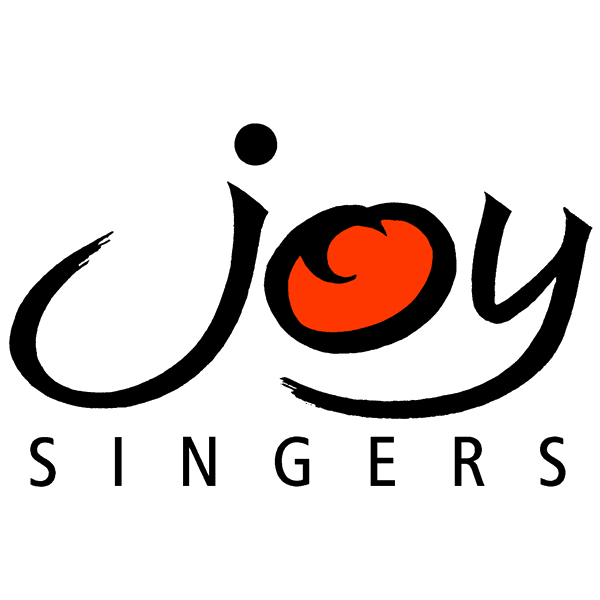The image features a company logo set against a completely white background. The logo consists of two words: "Joy" and "Singers." The word "Joy" is prominently displayed in the upper center in a very large, hand-painted black font, characterized by its irregular and swiftly drawn letters, with visible paint stroke ends. Notably, the O in "Joy" is distinctively filled with red and is drawn such that the ends of the circle overlap, enhancing its hand-drawn appearance. Below "Joy," the word "Singers" is presented in a smaller, uppercase, bold typeface. The use of black and red stands out against the stark white background, creating a simple yet striking logo likely designed for corporate branding, such as on a website, menu, or business card.